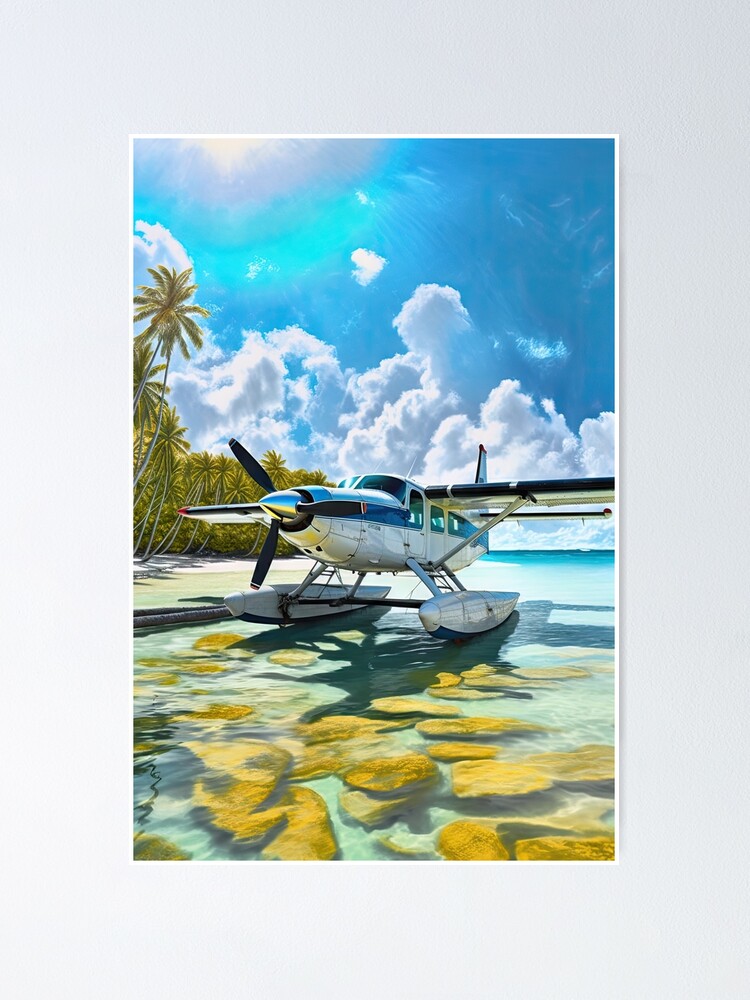This detailed and meticulously crafted image appears to be a painting of a seaplane gracefully resting on a shallow body of water. The seaplane, characterized by its sleek silver body complemented with blue highlights, stands prominently in the foreground. It features a three-bladed black rotor at the front and is positioned in such a way that it faces the left side of the image, casting a clear shadow on the transparent blue water beneath. The serene water allows the view of brown rocks through it, enhancing the scenic depth.

Above, the sky is an expansive, vibrant blue scattered with fluffy white clouds. The radiance of the bright sun, positioned in the top left corner, illuminates the scene, adding a warm hue to the tranquil environment. The presence of lush green trees on the left side, possibly coconut or palm trees, adds to the tropical essence of the setting, their foliage vibrant against the blue sky and sandy beach.

This artwork, possibly digitally created or a traditional painting, presents a vivid daytime scene by the beach. The main composition sits within a white-bordered grey matte, emphasizing its rectangular format. The overall visual is detailed with colors including turquoise, aqua, and light gold, reflecting a harmonious balance of natural aquatic and sky elements. The seaplane, resting on white pontoons, is central to this idyllic seaside setting, creating a peaceful yet dynamic visual narrative.